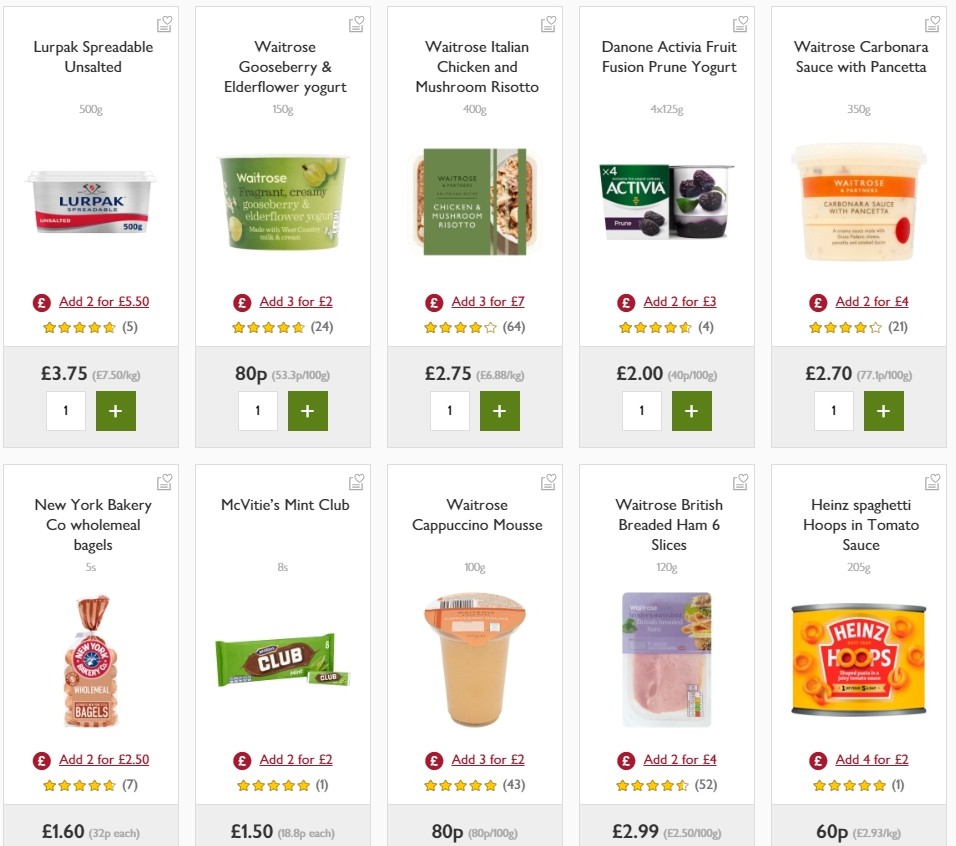The image consists of two panels, arranged vertically, with the top panel and bottom panel each being divided into two rows. In each row, there are five sections containing product details, each with a white top part and a gray bottom part.

**Top Panel:**
1. **Lur-Pak Spreadable Unsalted**
   - Image of the product
   - Offer: Add 2 for £5.50, or individually priced at £3.75
2. **Waitrose Gooseberry and Elderflower Yogurt**
   - Image of the product
   - Offer: Add 3 for £2.80
3. **Waitrose Italian Chicken and Mushroom Risotto**
   - Image of the product
   - Offer: Add 3 for £7.00, or individually priced at £2.75
4. **Danone Activia Fruit Fusion Prune Yogurt**
   - Image of the product
   - Offer: Add 2 for £3.00, or individually priced at £2.00
5. **Waitrose Carbonara Sauce with Pancetta**
   - Image of the product
   - Offer: Add 2 for £4.00, or individually priced at £2.70

**Bottom Panel:**
1. **New York Bakery Co. Wholemeal Bagels**
   - Image of the product
   - Offer: Add 2 for £2.50, or individually priced at £1.60
2. **McVitie's Mint Club**
   - Image of the product
   - Offer: Add 2 for £2.00, or individually priced at £1.50
3. **Waitrose Cappuccino Mousse**
   - Image of the product
   - Offer: Add 3 for £2.80
4. **Waitrose British Breaded Ham (6 slices)**
   - Image of the product
   - Offer: Add 2 for £4.00, or individually priced at £2.99
5. **Heinz Spaghetti Hoops in Tomato Sauce**
   - Image of the product
   - Offer: Add 4 for £2.00, or individually priced at 60 pence